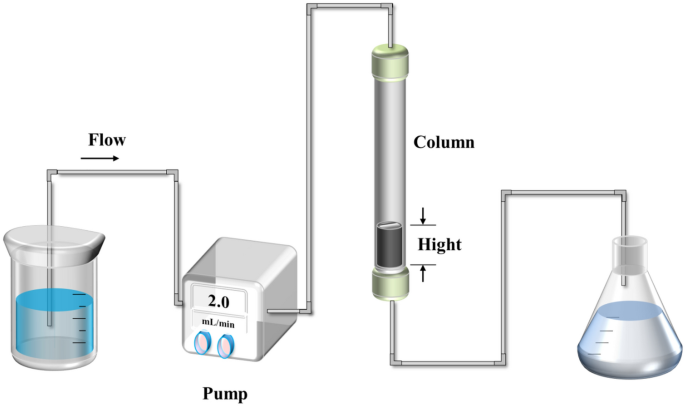The diagram appears to be from a textbook, illustrating a chemical process. It starts on the left with a graduated cylinder filled with water, indicated by notches. Connected to this is a pipe that extends upwards, turns right at a right angle, and then downwards. Above this pipe, the word "flow" in black font is accompanied by a right-pointing arrow. The pipe leads to a white pump labeled "2.0 milliliters per minute," featuring two knobs. From the pump, the pipe continues, ascending, turning right, descending, to connect to a cylindrical tube labeled "column" and "height." The interior of this column appears to contain a dark material, potentially a liquid or solid. The pipe continues its path, going downwards, then right, up, right, and down again to reach another beaker at the far right. This final beaker has a pyramid shape and is filled with a grayish-blue liquid.